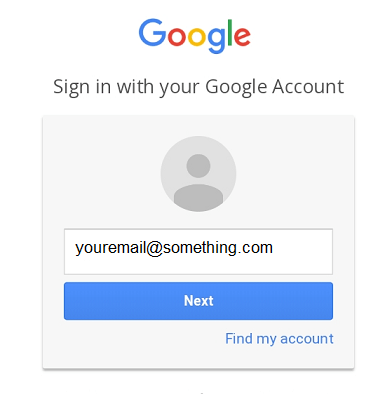This image is a detailed screenshot of a Google sign-in page. The screenshot prominently features the Google logo at the top, which is depicted in its iconic colors: blue, red, yellow, blue, green, and red. Below the logo, the phrase "Sign in to your Google Account" is written in gray text.

Central to the image is a light gray sign-in box that appears slightly shaded, giving it a three-dimensional effect. Inside this box, there is a gray circle containing a silhouette of a person, symbolizing account identity.

Below the circle, placeholder text reads "your email at something.com." At the bottom of the box, a blue button with white text reads "Next," indicating the option to proceed with the sign-in process. Underneath this button, "Find my account" is written in blue text, providing an additional account recovery option.

The image overall is clean and simple, designed to guide users through the sign-in process for their Google account.